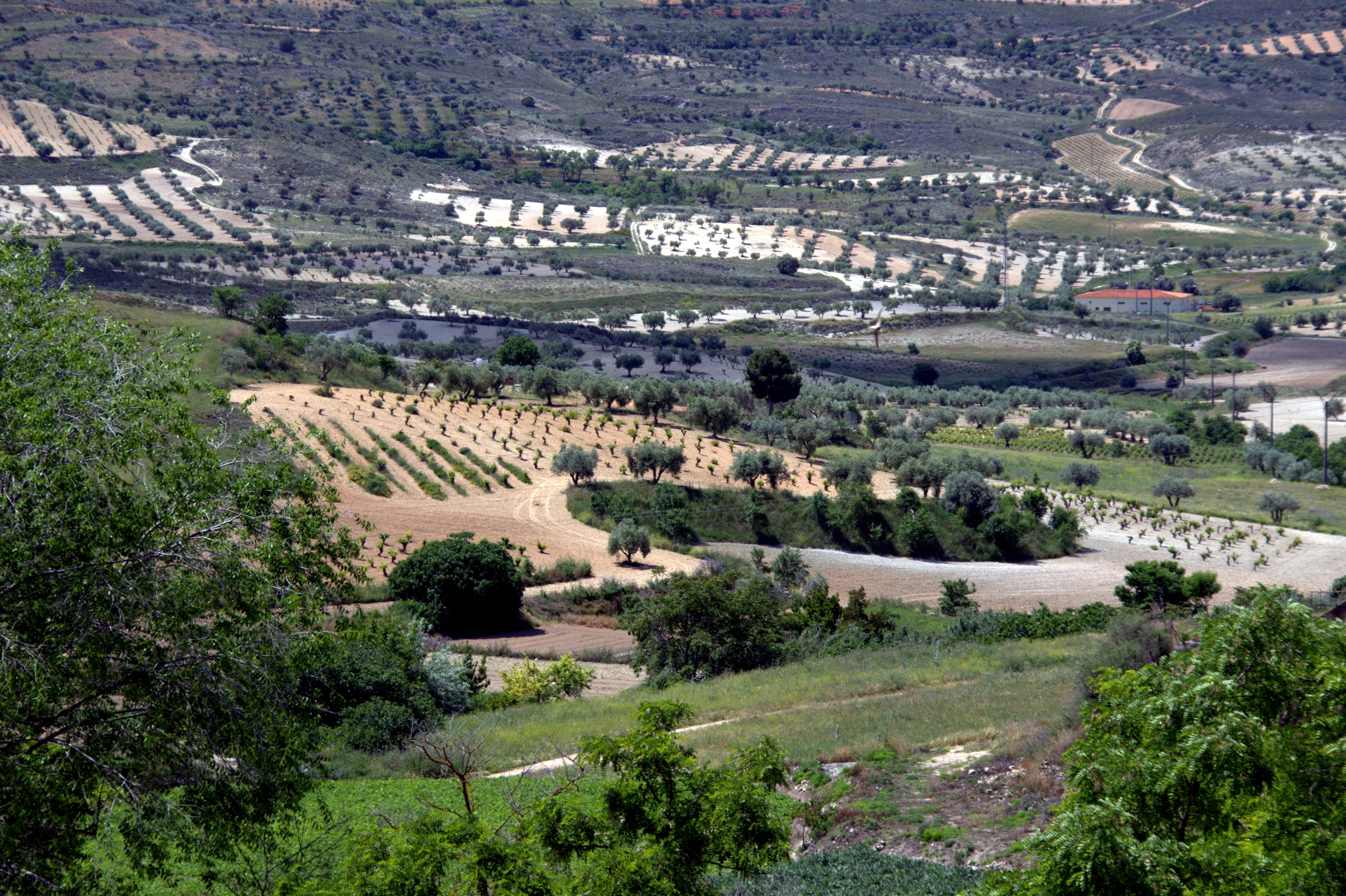This aerial photograph, likely captured from a drone or airplane, showcases a sprawling agricultural landscape composed of various plots of farmland against a hillside. Dominating the scene are rows of verdant crops, possibly orchards or vineyards, organized in meticulously cultivated patterns. In the lower foreground, leafy green canopies, akin to tall trees or shrubs, delineate the edge of a grassy field bordered by hedge rows. Behind this, a distinct circular area of neatly aligned vegetation suggests intensive cultivation, possibly of vines or olive trees. The midsection of the image features an oval patch of densely growing trees, indicating another cultivated area. The terrain seems to incline slightly, leading to additional stretches of land with crops planted in vertical and horizontal rows. A dirt road or perhaps a creek runs through the meadow below, contributing to the region's intricate layout. Scattered bushes and trees add to the natural tapestry. The image, rectangular in shape and devoid of a visible horizon, immerses the viewer in the full, lush splendor of late spring or summer agriculture.